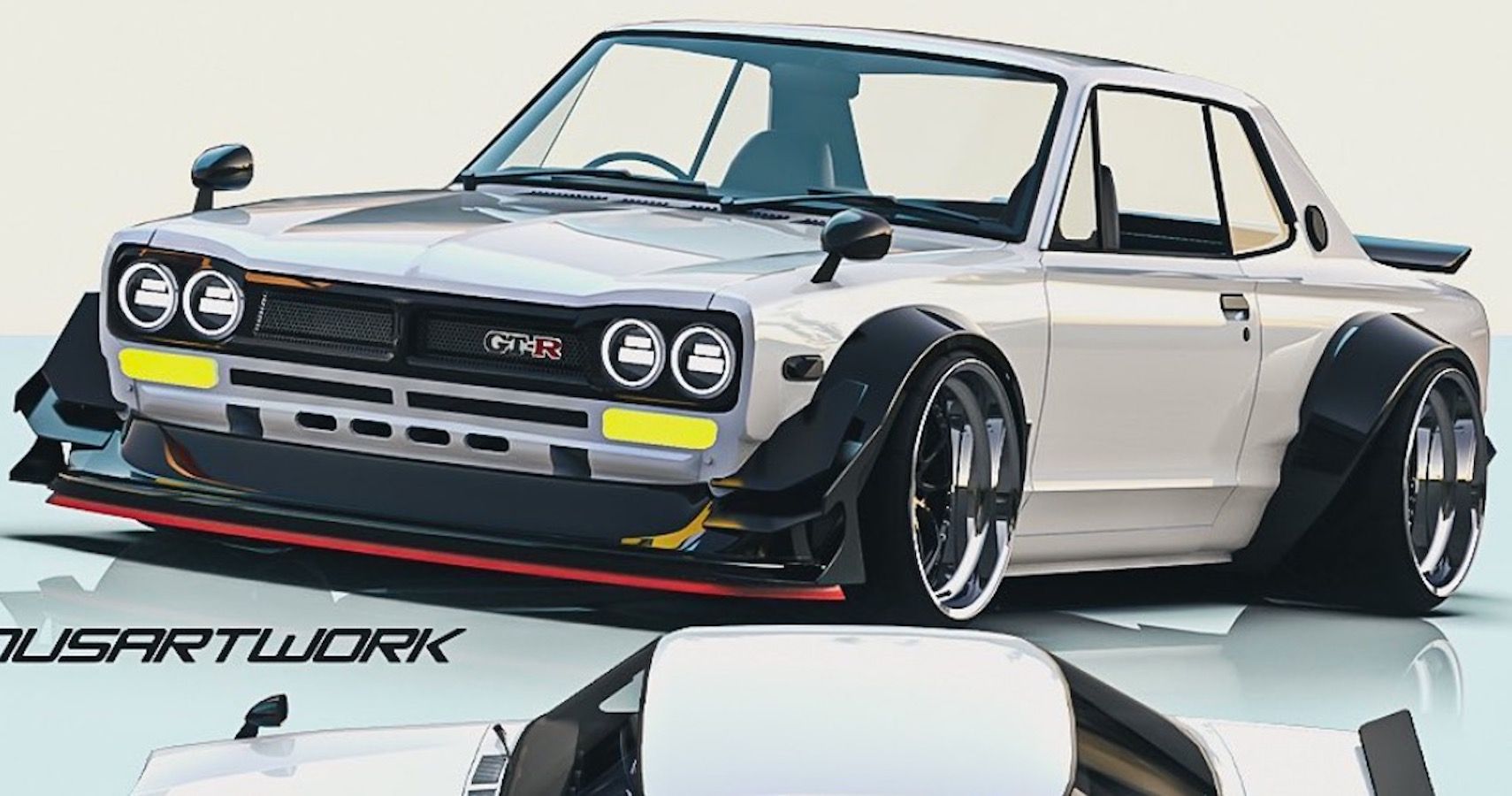This detailed color photograph is likely promoting the GT-R race car, capturing its sleek design and prominent features. The primary image showcases a low-slung, two-door coupe in light gray, situated on a reflective light blue surface, with an off-white or very light gray background. The car's wheels are large racing wheels that extend beyond the fenders but are partially covered by black metal extensions, forming part of the black trim that complements the white body. The front of the car boasts a large black grille adorned with two circular yellow structures, likely lights, on each end. The grille bears the GT-R logo, with "GT" in black and "R" in red letters. Further accentuating its sporty profile, the car has black side view mirrors mounted on the front fenders and a black rear spoiler.

The image also includes an overhead view of the car, focusing on the roof and integrated into the lower section of the main photograph. The positioning of these two car images is central, providing a comprehensive view of the vehicle's design and features. Text appearing in the lower left side of the image is partially visible, stating "US Artwork" and "SART work," suggesting the promotional or artistic nature of this piece.